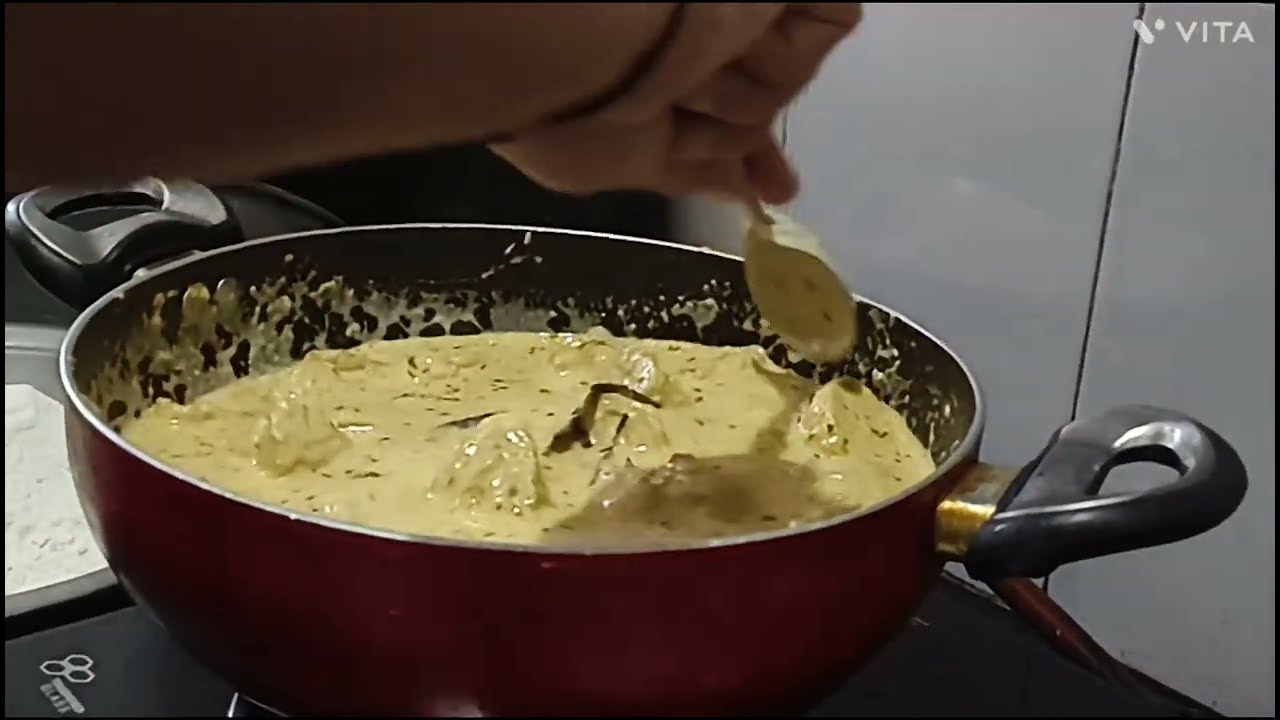The image showcases a close-up of a red, shallow skillet with rounded edges and dual short black handles, resembling a pot. Inside, there's a creamy, yellowish, cheesy dish with visible chunks of chicken and specks of parsley-like herbs. A person's hand, emerging from the top left of the frame, is seen holding a spoon, poised to stir the contents. The skillet is set against a gray wall background. In the top right corner, the logo "Vita" suggests it could be a cooking show. To the left of the skillet, there's a small tray of what appears to be flour.